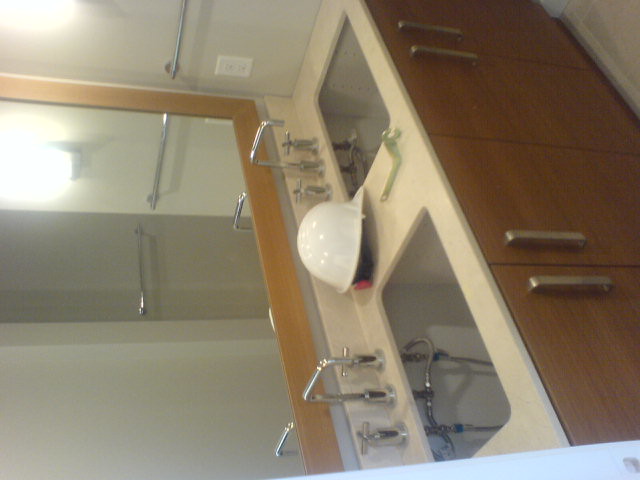This image showcases a kitchen vanity featuring a double sink, though it's depicted sideways, which might make it slightly disorienting. On the left side of the vanity, there is a large mirror framed in rustic, weathered wood. A white hard hat rests on the pristine white countertop, accompanied by a black strap with a red backing underneath it. In the center space between the two sinks lies a wrench, emphasizing an unfinished setup. The double sinks themselves lack their basins, with exposed plumbing visible underneath, though stainless-steel faucets are already installed. The vanity is adorned with a rich brown wood trim, featuring long, vertical metallic handles. A light source reflected in the mirror appears to emanate from the direction of what is, due to the image's orientation, the top of the photo. The walls are painted in a subtle white-gray hue, while the floor sports a light brown tone, bringing warmth to the overall scene.